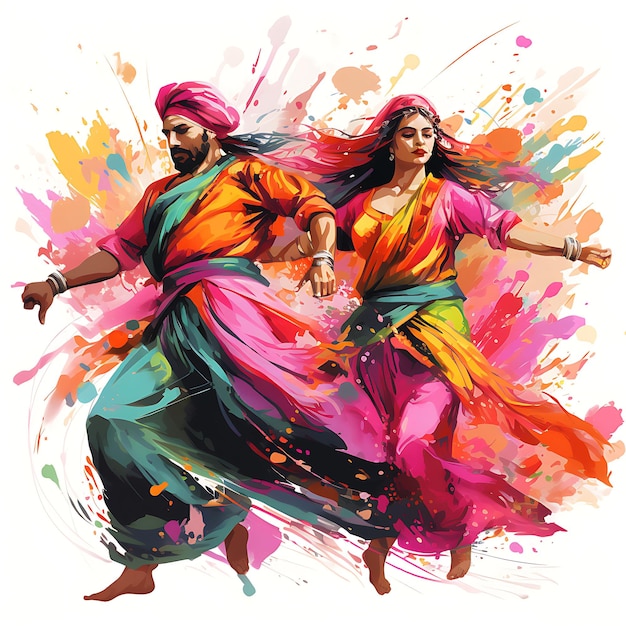This digital illustration features a vibrant scene set against a backdrop of warm-colored paint splatters, including shades of pink, light blush, red, orange, and muted teal, all on a white background. In the foreground, a man and woman, dressed in colorful traditional attire, are engaged in a dance. The man, positioned on the left, sports a pink head covering, a black beard, and a mustache. He is clad in an orange kurta and green dhoti, accessorized with a pink top cover and a waistband, and is barefoot. The woman, on his right, has long, flowing black hair and wears robes in warm tones with pops of teal, tied at the waist with a blue cloth. Both dancers adorn bangles on their wrists and have their sleeves rolled up to their elbows. The couple stands close together, facing the viewer with the woman's arm behind the man's back, enhancing the intimate and dynamic nature of their dance.